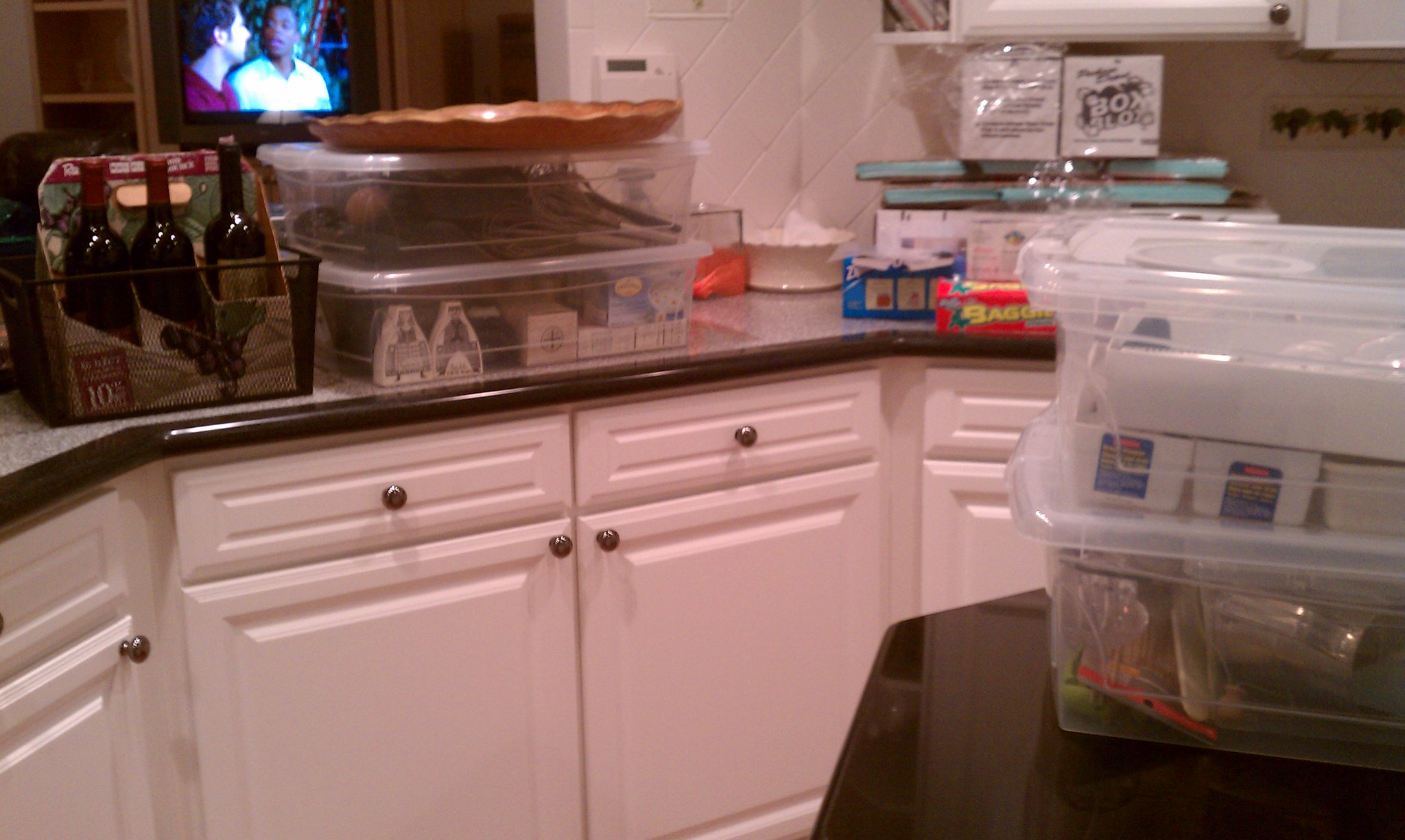In this image, we see a cozy kitchen setting with a television in the background displaying a scene featuring two actors – one Caucasian man in a white t-shirt and another, also Caucasian, wearing a purple shirt and standing to the left. On the grey and black speckled kitchen counter, which is accentuated by a brown outline at the front edge, lie three wine bottles. The two shorter bottles on the left sport red labels, while the taller one in the center features a cork and a distinctive design with a brownish base and grape illustrations.

The white shelving beneath the counter is stylishly detailed with white trim squares in a beveled formation. To the right, a plastic container rests on a black marble table. Just behind this, a white wall resembles a tiled surface extending to the right at an angle. A porcelain piece, indicative of a light fixture or thermostat, is mounted on this wall. Above and below the kitchen counter, we observe white cabinets adorned with elegant brass circular handles, consistent on both the drawers and cabinet doors.